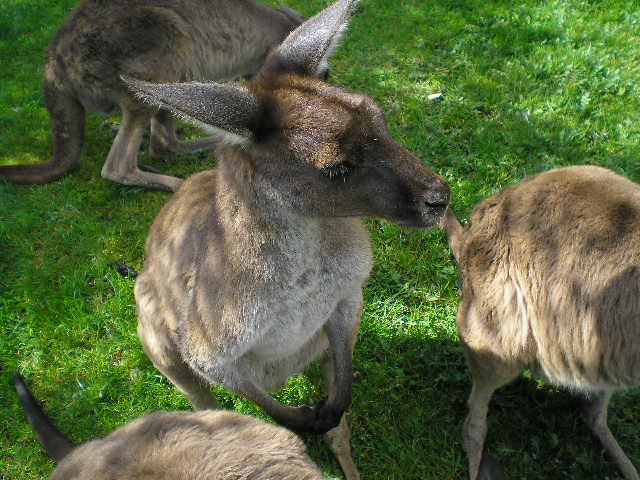This overhead photograph vividly captures a group of four kangaroos grazing on lush, bright green grass. The greenery forms a vibrant backdrop, emphasizing the kangaroos' multi-shaded brown fur. The central kangaroo, fully in frame, stands on its hind legs with its dark front paws slightly curved together, looking away from the camera. This kangaroo's body transitions from a dark tan and light brown on its back to a lighter, almost whitish hue on its neck and underbelly. Its face and muzzle are much darker, almost black, contrasting with the lighter, white insides of its ears. To the left, another kangaroo’s side is visible, its head lowered as if nibbling on the grass, with only its tail and part of its body visible. At the bottom, just an ear hints at another kangaroo's presence, while to the right, you can see the lower half of a fourth kangaroo, which has a more grayish tint to its fur. All kangaroos sport dark eyes, appear well-fed, and their fur looks pristine and well-maintained.